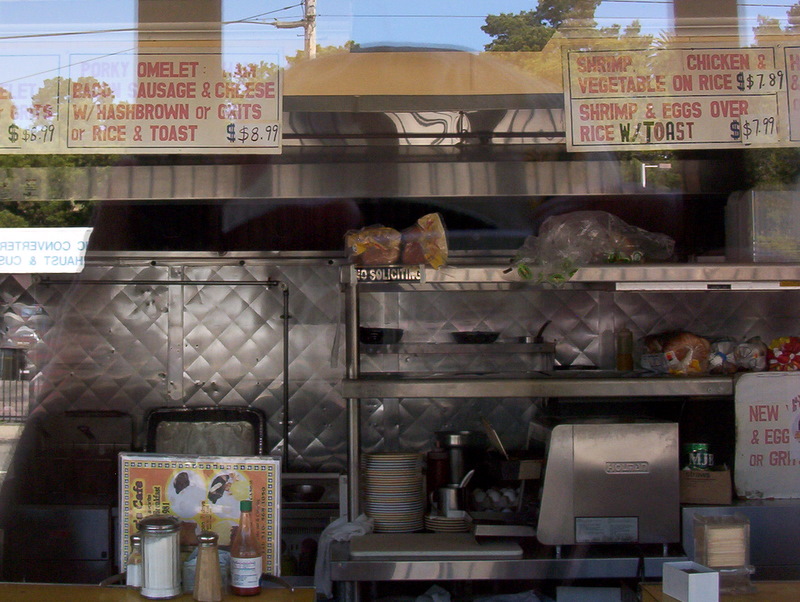The image is a color photograph showcasing a detailed view through a reflective glass window into a bustling restaurant kitchen. The window reflects a bright blue sky, leafy green trees, and power lines, adding a layer of complexity to the view. Inside, on the left side, there is a counter cluttered with condiments such as sugar, salt, pepper, and hot sauce, as well as an embedded menu amidst them. A stainless steel cabinet and shelves dominate the background, filled with loaves of bread, bags, and various kitchenware. Prominently placed behind the counter is a large stainless steel refrigerator. On the right, a monitor for a register can be seen. Above this scene, hanging menus with white backgrounds and red lettering detail the offerings: "Shrimp, chicken, vegetable, or rice $7.89," "Shrimp and eggs over rice with toast $7.99," and "Porky omelet with bacon, sausage, cheese, hash brown or oats or rice and toast $8.99." The menus feature additional listings that are partially obscured. The overall aesthetic is one of Photographic Representationalism Realism, capturing a precise and vibrant snapshot of the restaurant's interior.